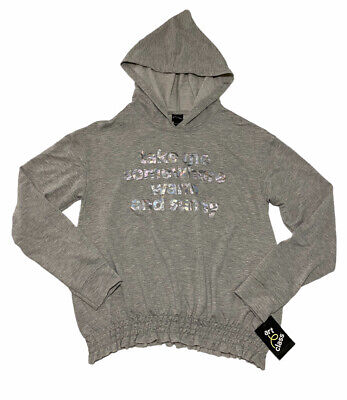This image depicts a gray hoodie pullover with long sleeves and a distinctive elasticized, shirred bottom hem, tailored likely for a female. The fabric features a intricate knitted cuff at the sleeves' ends. Notably, there is a black tag with white writing located near the cuff on the right sleeve; it possibly denotes the garment's brand or name and appears to read "art class." The hoodie bears partially legible, reflective silver-white text at the center, which might say "wake me something" or "take me somewhere" though it remains unreadable due to wrinkles and worn-off lettering. The overall color scheme of the garment is primarily gray with subtle black elements. Set against a plain white background, the hoodie is presented unworn, as if for a store advertisement, accentuating its details such as the wrinkled fabric and the unique ruffled appearance of its lower part.